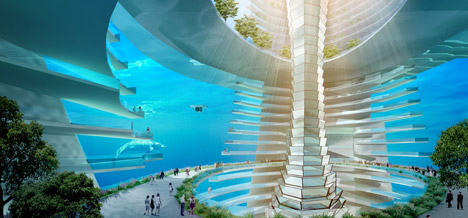The image depicts an intricate and immersive scene, seemingly inside a colossal, state-of-the-art aquarium. The background is dominated by a vast, ocean blue hue, lending an underwater ambiance. At the heart of the image is an imposing, cylindrical whirlpool structure that ascends from the ocean floor to the surface. The structure features alternating bands of white and steel gray, resembling a grand spine with rib-like extensions, giving it a futuristic and skeletal appearance. 

The top of this whirlpool-like tower reaches up to a cement-like edged opening, where sunlight pours in, hinting at an external environment with trees or shrubbery peeking around the perimeter. Darker sea green aquatic plant life can be seen in each corner of the image, enhancing the underwater effect. 

On closer examination, one can see small human figures around the base of the central column, emphasizing the enormous scale of the setting. These people seem to be exploring the multi-leveled aquarium surroundings, with pathways and viewing areas designed to offer various perspectives of the aquatic world. The structure is surrounded by lush green areas with trees, adding to the natural yet surreal atmosphere.

Encircling the scene is a transparent glass wall of the aquarium, revealing massive water bodies inside which swim majestic sea creatures such as dolphins and whales. The building's architecture, with its vast open spaces, sunlight filtering through the ceiling, and the grand central column, creates a sense of elegance and advanced design, making it a breathtaking and immersive experience for viewers.